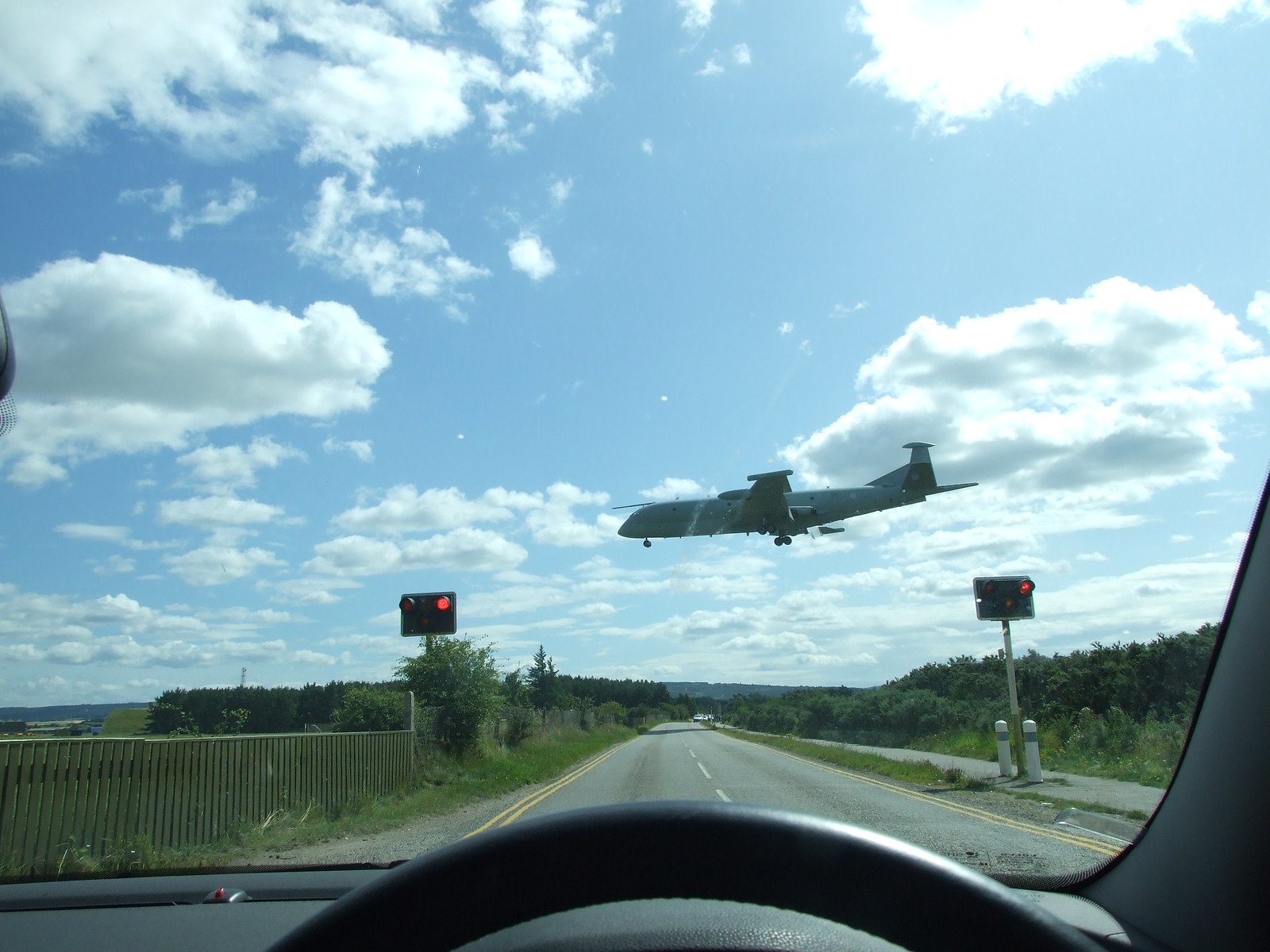A photograph taken from inside a car, likely using a cell phone or dash cam, captures a scene through the windshield. The image reveals part of the dark gray dashboard and the upper portion of the steering wheel. Prominently in the middle-right of the frame, an airplane is seen descending, with its landing gear extended, indicating it's preparing to land. The vehicle is stopped at a red traffic light, with the stoplight visible in the shot. It’s a bright day with scattered clouds, suggesting pleasant weather. The car is positioned on a two-lane road, and a strip of grass separates it from another road for oncoming traffic.